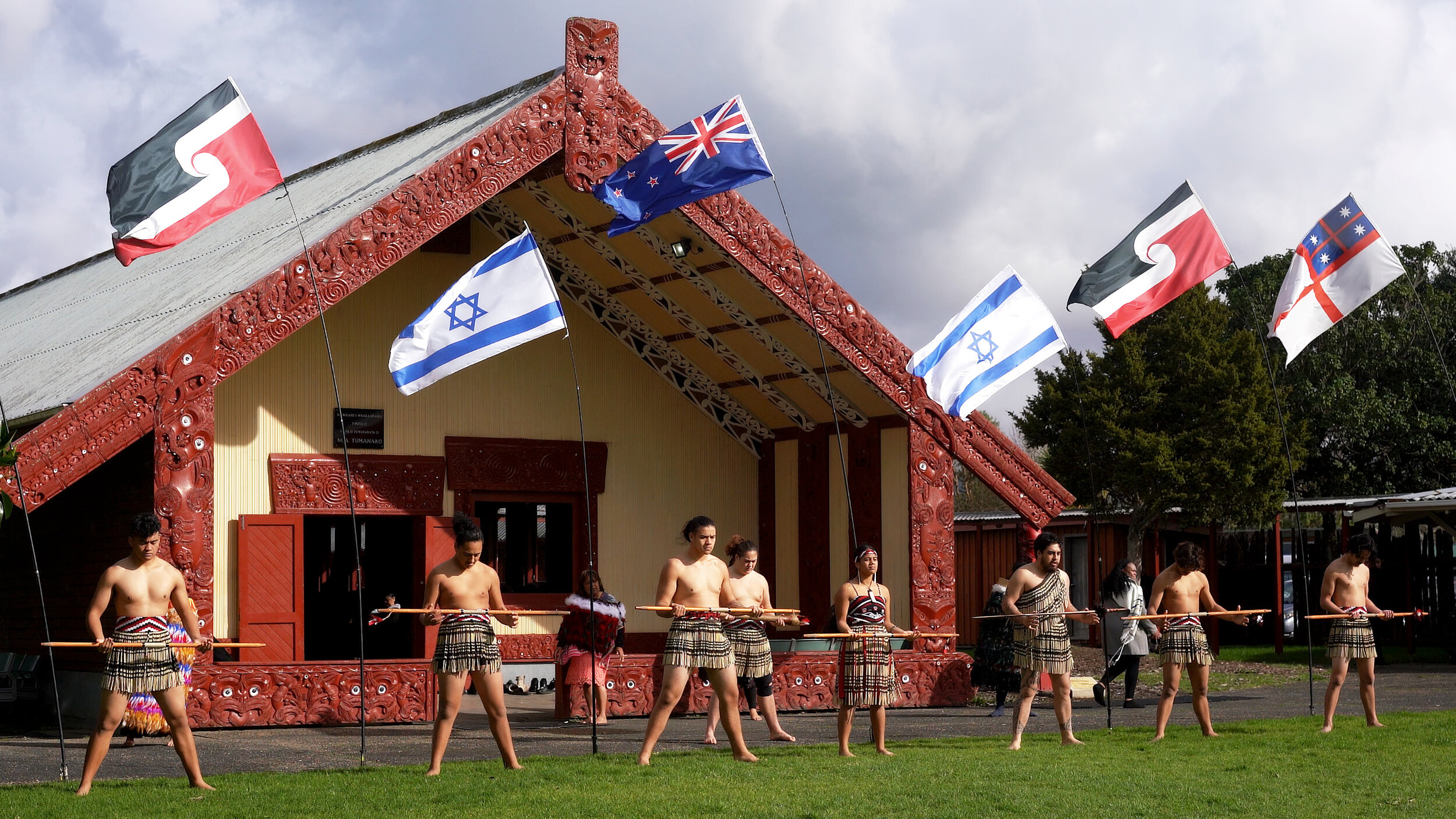This color photograph, oriented horizontally, captures a group of indigenous youth, predominantly male with one female, engaged in what appears to be a ceremonial dance or haka routine. The group, consisting of seven shirtless males donning skirt-like attire and a single female dressed similarly except for a tube-top, is positioned on a grassy lawn. Each participant holds a wooden staff or pole sideways, their legs spread in a traditional stance. Directly behind them stands a one-story building, likely a cultural center, distinguished by its intricate Maori carvings on the roofline and wooden columns. Flags fly above them, including the Israeli, Australian, and what appears to be variations of the Maori and British flags. The building features yellow walls and red trim, with additional low structures and tree shade visible in the background. Notably, one male wears a sash along with his skirt attire, differentiating him from the others.